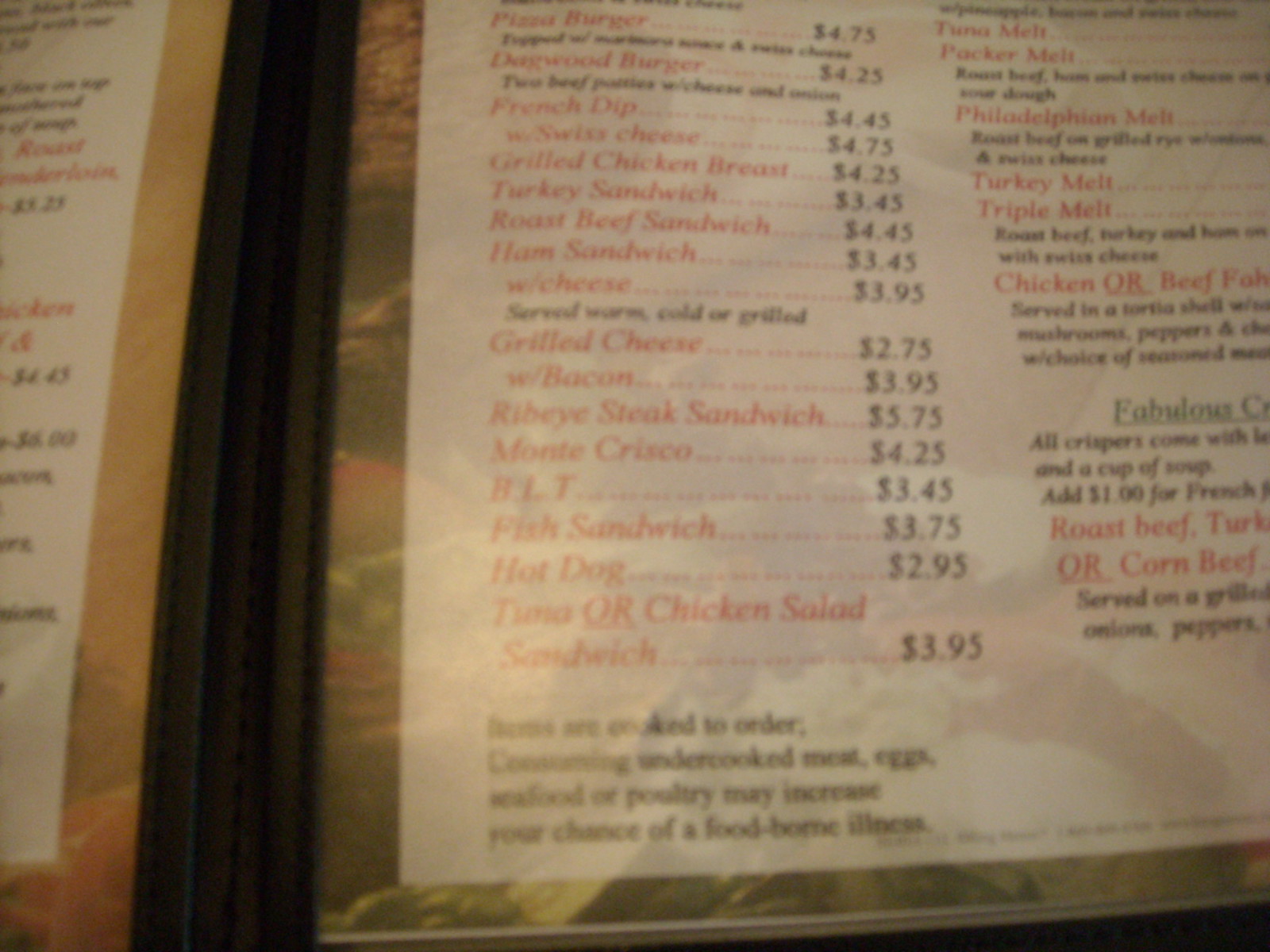This close-up image displays a menu featuring various mouth-watering food items. Each food item is elegantly listed in red font, while the prices are distinctively marked in black font. The menu includes:

- Plaza Burger: $4.75
- Dogwood Burger: $4.25
- French Dip: $4.45
- Swiss Cheese Burger: $4.75
- Grilled Chicken Breast Sandwich: $4.25
- Turkey Sandwich: $3.45
- Roast Beef Sandwich: $4.45
- Ham Sandwich: $3.45
- Grilled Cheese: $2.75
- Ribeye Steak Sandwich: $5.75
- BLT: $3.45
- Hot Dog: $2.95
- Tuna or Chicken Salad Sandwich: $3.95

Additionally, the menu offers specialty melts, including:

- Tuna Melt
- Philadelphia Melt
- Turkey Melt
- Triple Melt

Each item is presented clearly, making it easy to choose from a variety of delicious options.